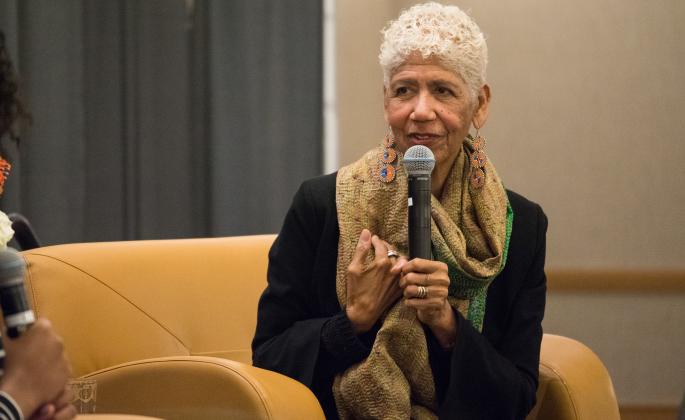This detailed image captures an older woman with short, very curly white hair, sitting in a smooth, wide, tan pleather chair. She is engaged in what appears to be a talk show or panel discussion, suggested by her poised microphone-holding stance. Her medium skin tone contrasts sharply with her black long-sleeve top and the striking gold and green scarf looped around her neck, which features intricate green detailing prominently on the right side. 

Elaborate earrings adorn her ears; these earrings are tiered medallions that dangle down to her shoulders, with mismatched elements that include blue and orange hues. Her right hand, slightly raised toward her chest, suggests an engaged and active presence in the conversation. The setting includes a gray curtain on the left side of the backdrop, transitioning to a tan wall on the right. Off to the right, barely within the frame, is another individual with curly black hair and a tan hand clutching a microphone, further indicating a shared moment of discussion. The overall atmosphere is intimate and focused, enhanced by the muted tones of the background and the smooth texture of the chair.